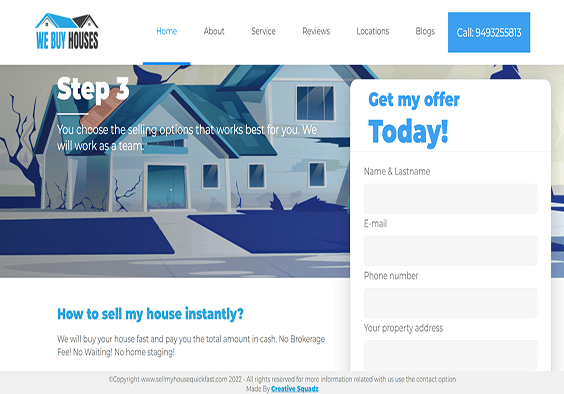This is a cropped screenshot of the WeBuyHouses website. 

At the top left, there's the WeBuyHouses logo. To the right, the header features several categories: "Home" (highlighted), "About," "Service," "Reviews," "Locations," and "Blogs." A blue box on the far right displays a contact number in white text.

Beneath the header, a large image of a deteriorating house is prominently featured, with significant cracks and signs of disrepair. Overlaid on the left side of the image is the text: "Step 3. You choose the selling options that work best for you. We will work as a team."

At the bottom left of the image, light blue text reads: "How to sell my house instantly," and below that, additional text states: "We will buy your house fast and pay you the total amount in cash. No brokerage fee, no waiting, no home staging."

On the right side of the image, there is a large overlay box with a prompt: "Get my offer today," with "today" written in very large letters. This box includes fields for "Name," "Last Name," "Email," "Phone Number," and "Your Property Address."

At the very bottom of the screenshot, a gray bar includes a copyright notice that states, "© [Year] WeBuyHouses. All rights reserved," followed by "Made by Creative Studios" in a blue hyperlink.